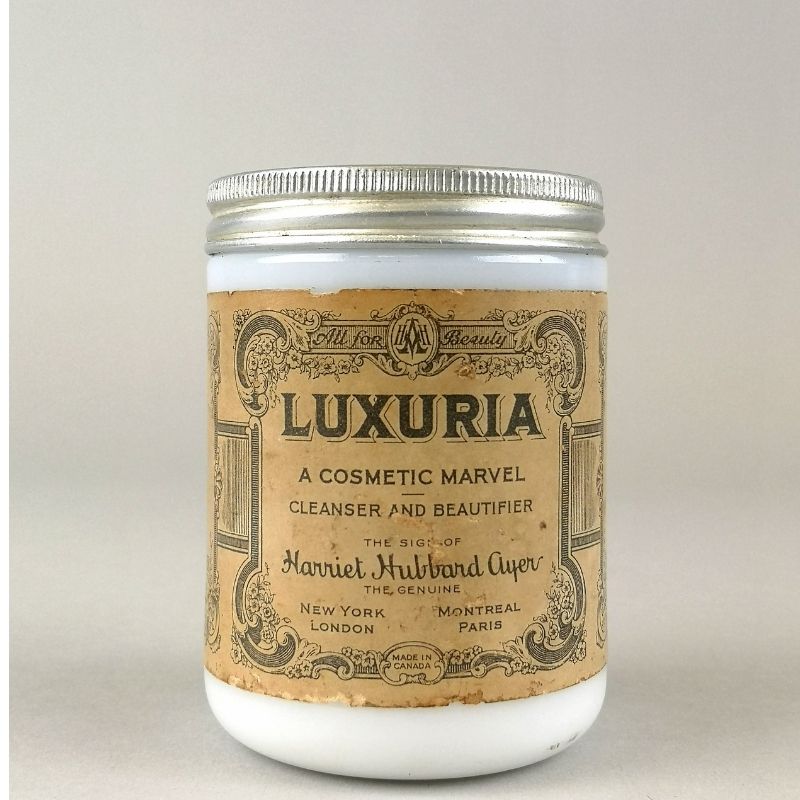This image showcases a vintage glass jar of cosmetic cream, prominently set against a gray background, reminiscent of a product shot for a website. The clear jar, which takes up about 70-80% of the image, features a silver screw-top lid. Inside, the jar contains a white lotion or cream. The center of the jar is adorned with an ornate, old-fashioned brown label that adds to its antique appeal. The label proudly displays "All For Beauty" at the top, followed by "Luxuria, a cosmetic marble cleanser and beautifier." Below this, in an elegant script framed with intricate scrollwork, it states "The sign of Harriet Hubbard Eyre, the genuine," and lists multiple prestigious locations: New York, London, Montreal, Paris. The label further notes that the product is "Made in Canada." The sophisticated design and vintage aesthetic suggest a luxurious, time-honored brand, possibly from the 1910s or 1920s.